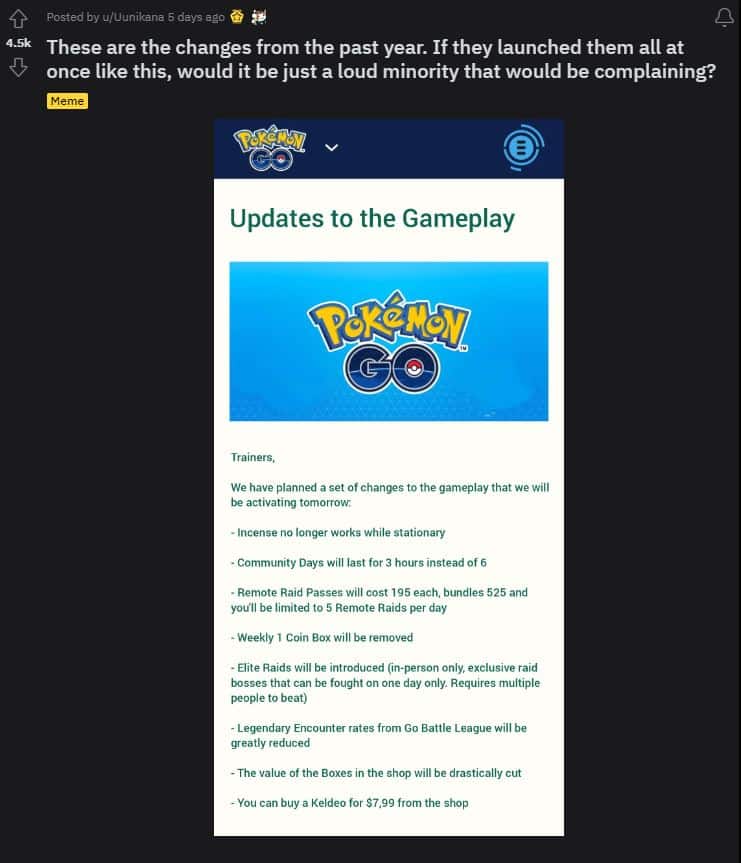The image is a detailed screenshot from Reddit, the online social community platform. The Reddit post is titled, "These are the changes from the past year. If they launched them all at once like this, would it be just a loud minority that would be complaining?" 

Embedded within the post is a secondary screenshot from the mobile game Pokémon Go. Central to the second image is the Pokémon Go logo, framed by a list of significant gameplay updates:

1. **Incense Effectivity**: Incense will no longer work while stationary.
2. **Community Days**: Community days' duration will be reduced from six hours to three.
3. **Remote Raid Pass Pricing**:
   - Individual Remote Raid Passes will cost 195 Pokécoins each.
   - Bundles of three will be priced at 525 Pokécoins.
   - Trainers will be limited to participating in five remote raids per day.
4. **Weekly Box Removal**: The weekly 1-Pokécoin box will be discontinued.
5. **Introduction of Elite Raids**: New Elite Raids will be added to the game.
6. **Decreased Encounter Rates**: The encounter rates for Legendary Pokémon from the Go Battle League will be significantly reduced.
7. **Box Value Reductions**: The in-game shop boxes will have their value drastically decreased.
8. **Keldeo Purchase**: Players will have the option to buy the mythical Pokémon Keldeo for $7.99 from the in-game shop.

The concise yet detailed list of changes captures the reader’s attention, sparking discussion on the impact and reception of these numerous updates within the Pokémon Go community.